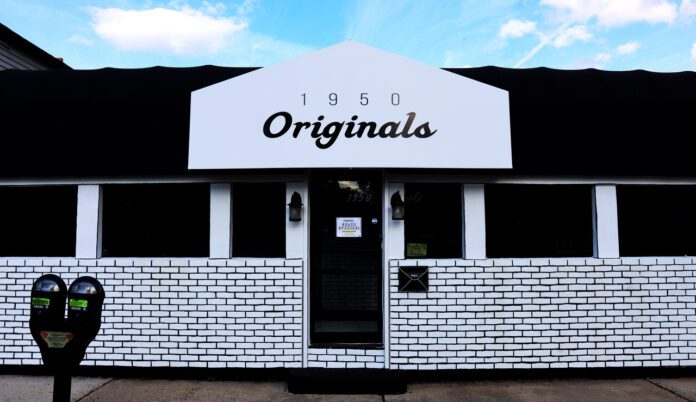This photograph captures the front exterior of a vintage storefront, potentially a retro-themed restaurant or business, accentuated by its classic design elements. The lower half of the façade is constructed from white brick with stark black mortar, while a series of large windows dominate the middle section, interspersed with white wall pillars. Centrally located is a substantial glass door framed in black, flanked by distinctive hanging globe light panels. Above the windows, a black corrugated surface doubles as an awning, ornamented with a long, narrow pentagonal banner proclaiming "1950 Originals" in black cursive text. The scene is set against a background of a blue sky dotted with small, fluffy white clouds. In the foreground, a gray sidewalk and a black parking meter positioned to the left hint at a street running alongside this evocative storefront.